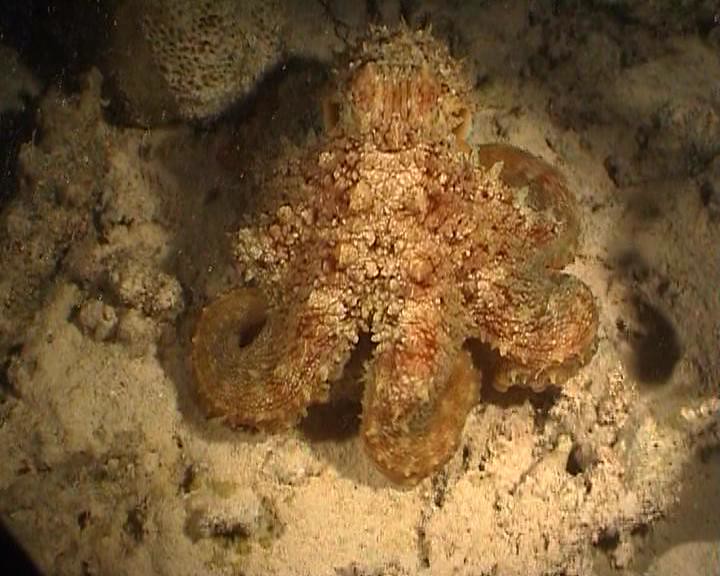This photograph captures a camouflaging sea creature, likely an octopus or a squid, nestled on a sandy, rocky ocean floor. The creature, which exhibits varying shades of orange and brown and a bumpy skin texture, is purposefully blending into its surroundings. Its body features a round, oval head with faint, darkly outlined eyes on either side. The tentacles of the sea creature, numbering at least four and appearing rubbery and flexible, are curled and tucked beneath its body, forming a star-like shape. The sandy background includes grains and pieces of tan coral, enhancing the creature's camouflage. This remarkable shot highlights the seamless integration of the creature into its natural habitat.